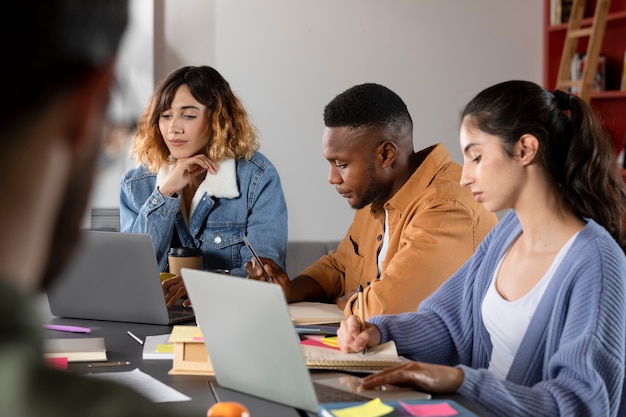In this stock photo of a group of young professionals in a casual office setting, three central figures are seated at a table with laptops, notebooks, and various stationery items like pencils, pens, and Post-it notes scattered around. The woman to the left, dressed in a denim jacket with a fleece collar, has medium-length curly hair that is dark at the roots and blonde at the ends. She is focused on her laptop screen, a coffee cup placed near her. Next to her, there is a black male with short-cropped hair, wearing a mustard-colored shirt over a white tee. He is concentrating on the notebook in front of him, holding a pen in his right hand. The third individual, a woman with long dark hair tied back in a ponytail, is clad in a cornflower blue ribbed cardigan over a white tank top. She is writing in a ruled notebook while her silver laptop remains open beside her. In the blurred foreground, there’s a partial glimpse of a fair-skinned man with a beard and glasses, likely the lecturer or another participant. The background of the room features a bookshelf equipped with a ladder, reinforcing the professional nature of the setting. The overall ambiance suggests a collaborative meeting or study session filled with focused attention and casual attire.